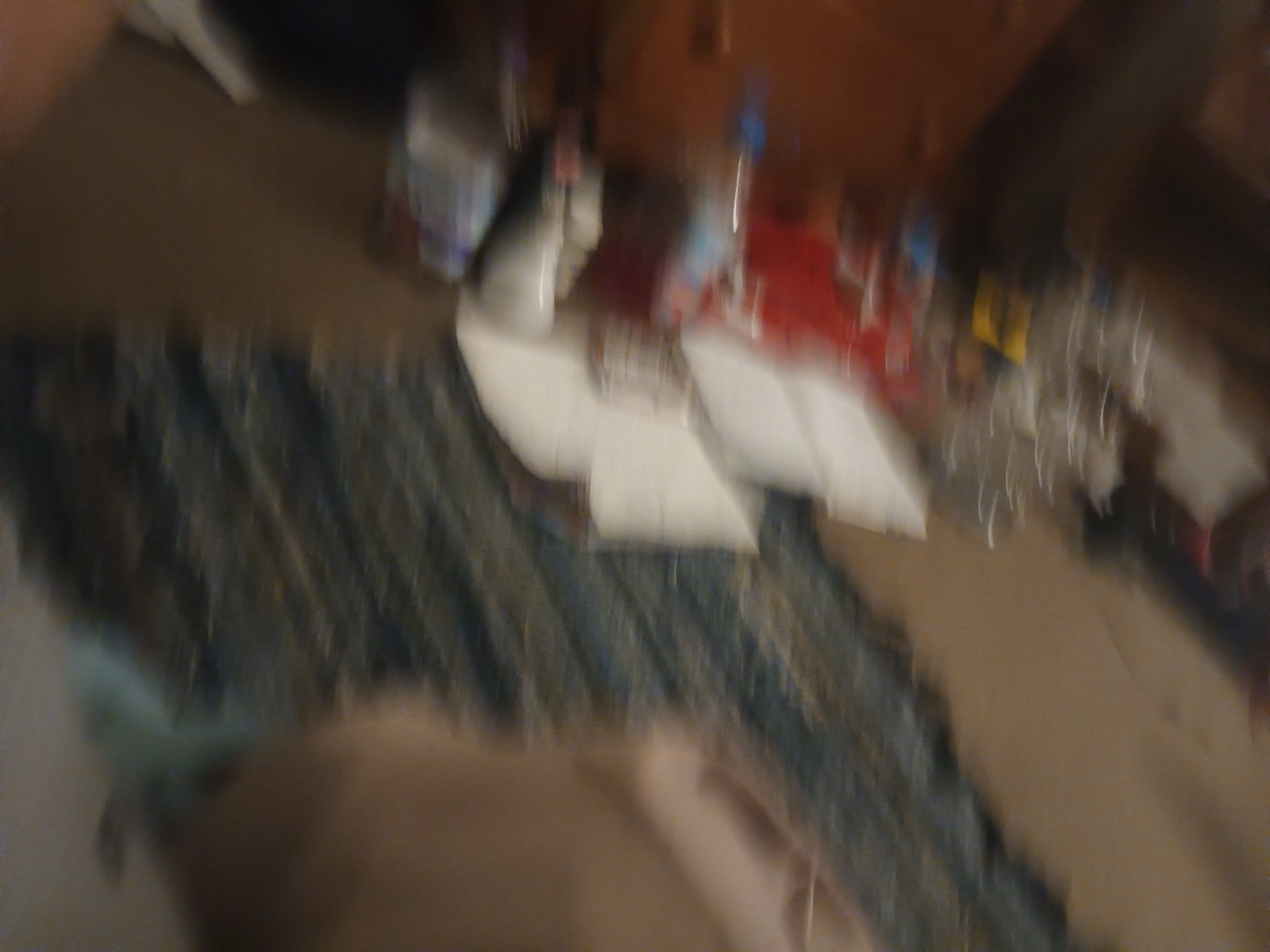This is a blurry colour photograph taken indoors, with a dominant brown and gray color palette. The foreground features the head and ears of a dog, suggesting it might have bumped the person taking the photo or is wearing a harness with a GoPro-like camera. The scene shows a cluttered room with a rectangular rug, shaded in grey, blue, and light blue tones, laid out with its longest side running away from the viewer. Scattered across the floor are assorted items including paper pads encroaching onto the rug, various bottles -- one appearing to be a drinks bottle with blue labelling and caps, another resembling a spray cleaning bottle -- and potentially a food package. Additionally, there are some red items and the base of a brown chair in the background, with empty bottles nearby. The upper regions of the image are marked by a mix of solid brown and reddish-brown hues, while the center contains a white object, possibly plastic, outlined sharply even in the blur, resembling stacked rectangular prisms with some red and grey elements that may be feathers or fabric.